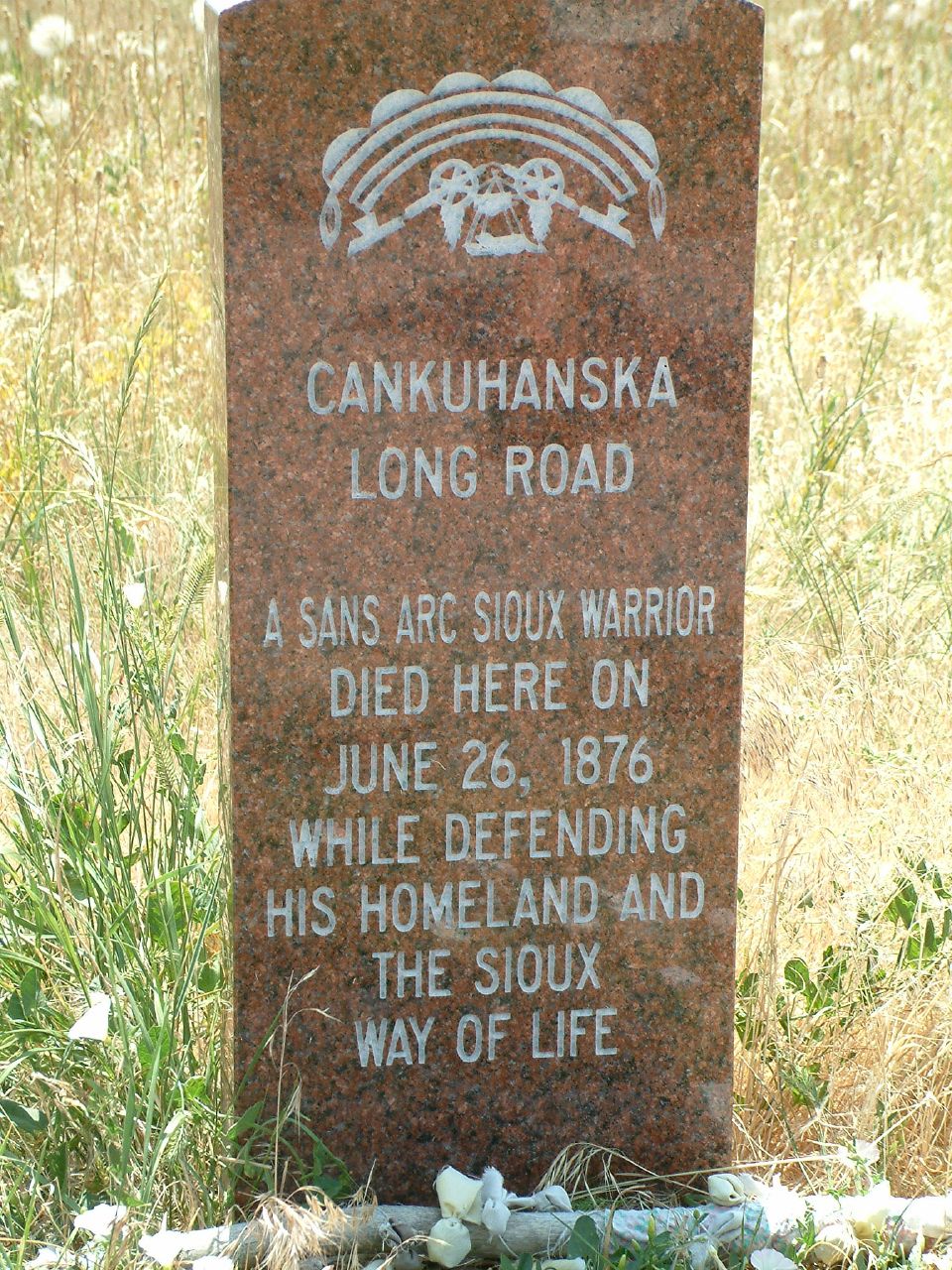The image depicts a red granite headstone set against a backdrop of green and yellow-brown grass and dotted with white wildflowers, suggesting a field in the Midwest on a sunny day. The headstone is rust-brown in color, speckled with black and white, and has a polished surface. At the top, an indistinct tribal symbol is etched into the stone. Below the symbol, the inscription reads: "Kankahanska Long Road." Beneath this, an epitaph states, "A Sans Arc Sioux warrior died here on June 26, 1876, while defending his homeland and the Sioux way of life." At the base of the headstone, a long white stick or branch lies on the ground in the shadow. The scene around the monument is marked by various grasses, some appearing dehydrated, and white puffy dandelions.